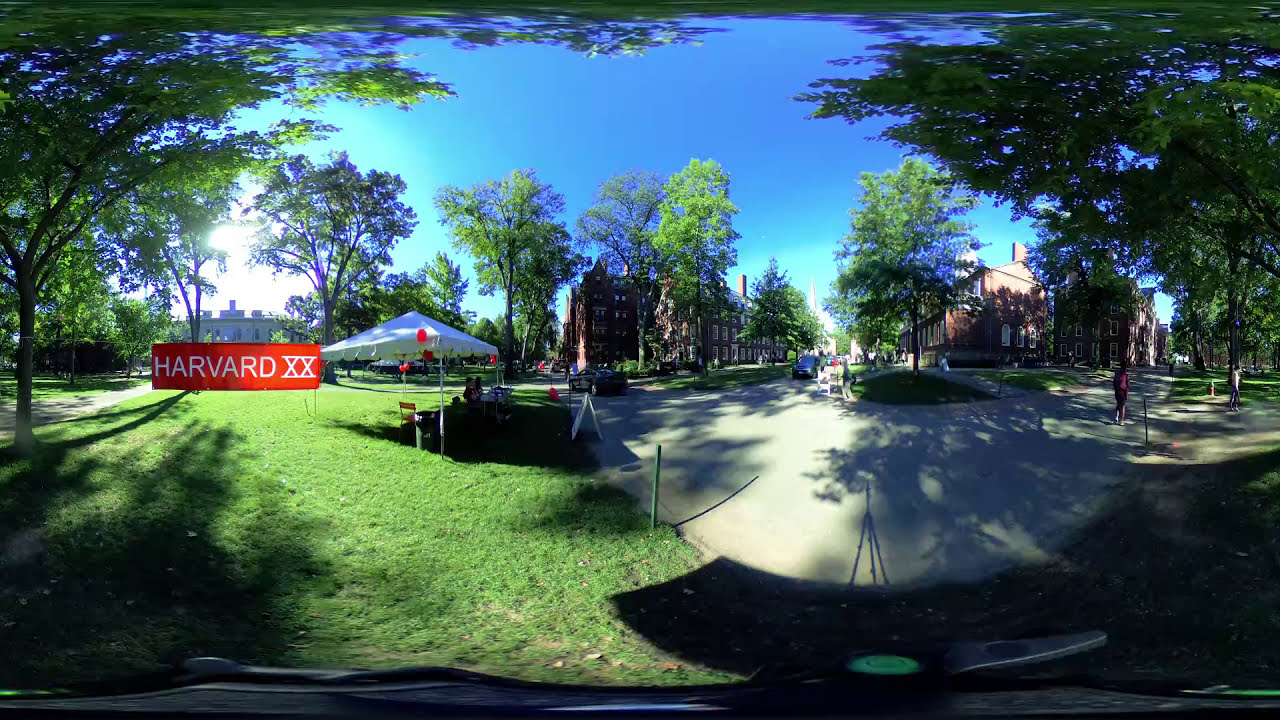This vibrant, wide-angle photograph captures the bustling and picturesque atmosphere of Harvard University's campus. The scene is dominated by a vivid green lawn, encircled by a cement walkway that connects the various historic, red-brick buildings, each standing three to four stories tall. Blue skies without a cloud in sight provide a stunning backdrop, with mature trees adding a touch of nature's beauty to the academic setting. 

Prominent in the image is a red-and-white sign reading "Harvard XX," firmly staked into the grass, further accentuating the educational prestige of the location. Adjacent to the sign, a small white gazebo serves as a focal point for campus activities, perhaps a recruitment or information station. Scattered across the scene are groups of students and other individuals, strolling or engaging with the tent, suggesting a lively, communal atmosphere. In the background, cars traverse a concrete road, adding a layer of urban dynamism to this serene academic enclave. The overall scene exudes traditional collegiate charm coupled with an inviting, active campus life.